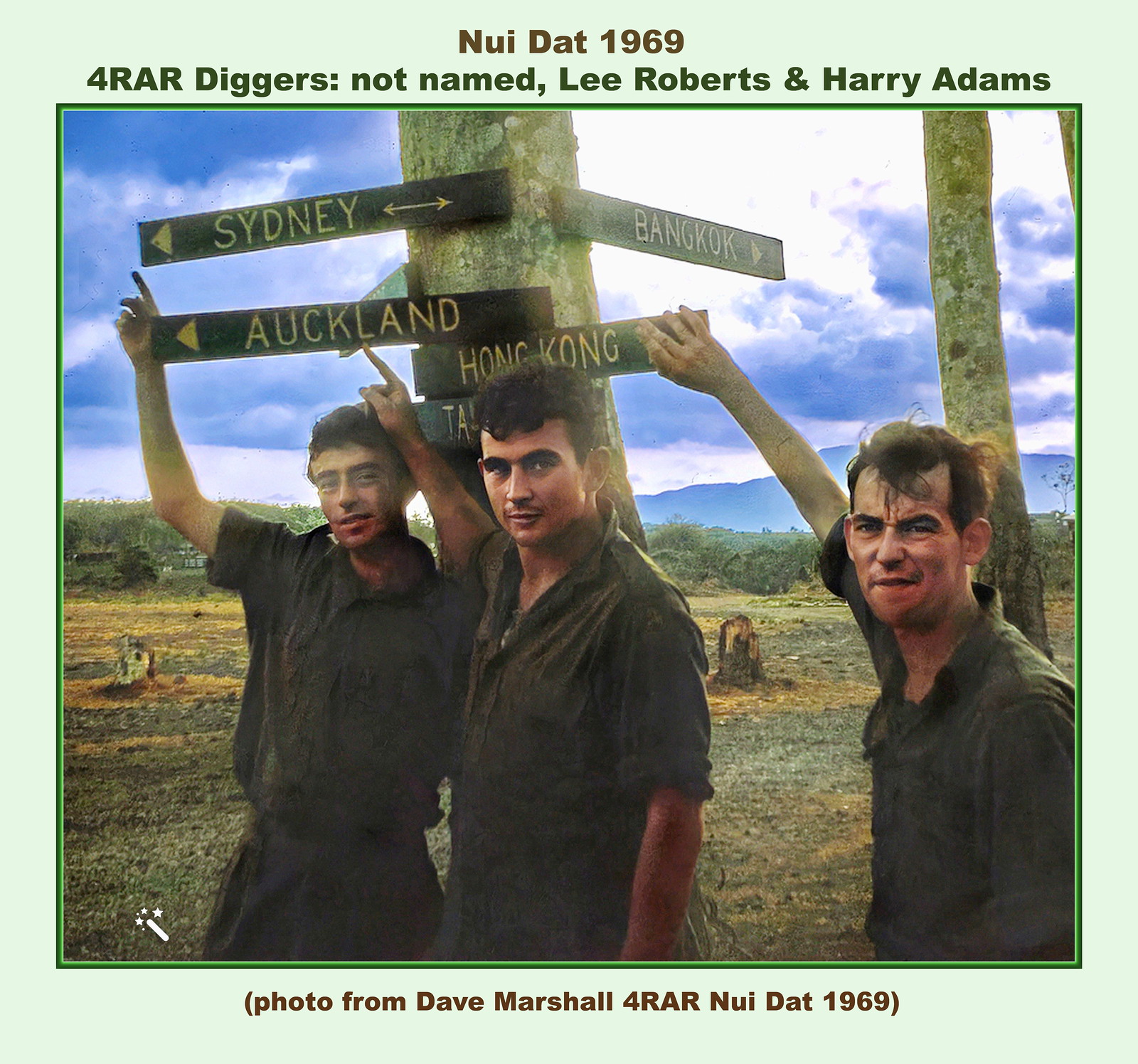The photograph, taken outdoors during the daytime, features three young, uniformed Caucasian men standing in front of a tree adorned with directional signs. The scene is set against a backdrop of a clear sky with slight wisps of clouds and distant blue mountains. The men, all sporting short brown hair and dressed in navy green coveralls, stand under signs pointing to cities like Sydney, Auckland, Bangkok, and Hong Kong, all marked with yellow arrows. The man on the far right raises his right hand, while the man on the far left holds up three fingers. The background includes vibrant greenery, trees, and grass, with low hills or possibly a grove of trees stretching across the horizon. The signs on the tree bear locations and directions, and above them, a sign reads "Nui Dat 1969" with the text "4RAR Diggers, not named Lee Roberts and Henry Adams," attributed to photographer Dave Marshall. Overall, the image appears to capture a commemorative moment with a military context, possibly related to an operation or unit stationed in Southeast Asia.